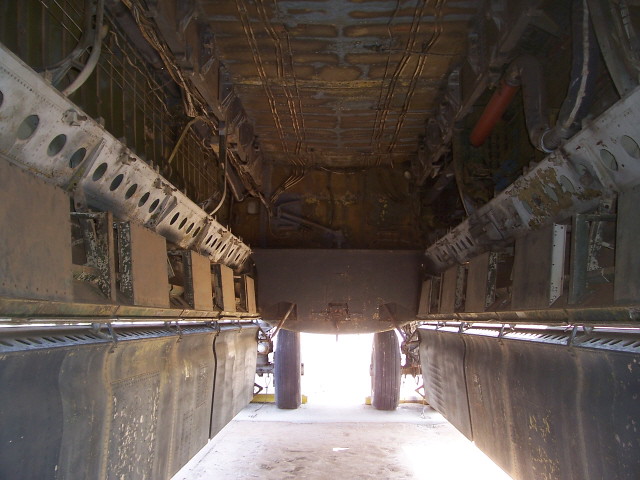The image depicts the rusty, dirt-laden undercarriage of a large, metal vehicle—most likely a semi-trailer or heavy-duty truck. Visible in the center are two wheels with axles, suggesting the photo was taken from a midway point. Along the sides, there are flaps that could potentially be for offloading cargo. The underbody is crisscrossed with a network of cable lines and large tubes, contributing to its complex mechanical structure. This vantage point underscores the vehicle's significant height and robustness, indicative of its heavy-duty nature, possibly designed for tasks like hauling construction materials or clearing snow.